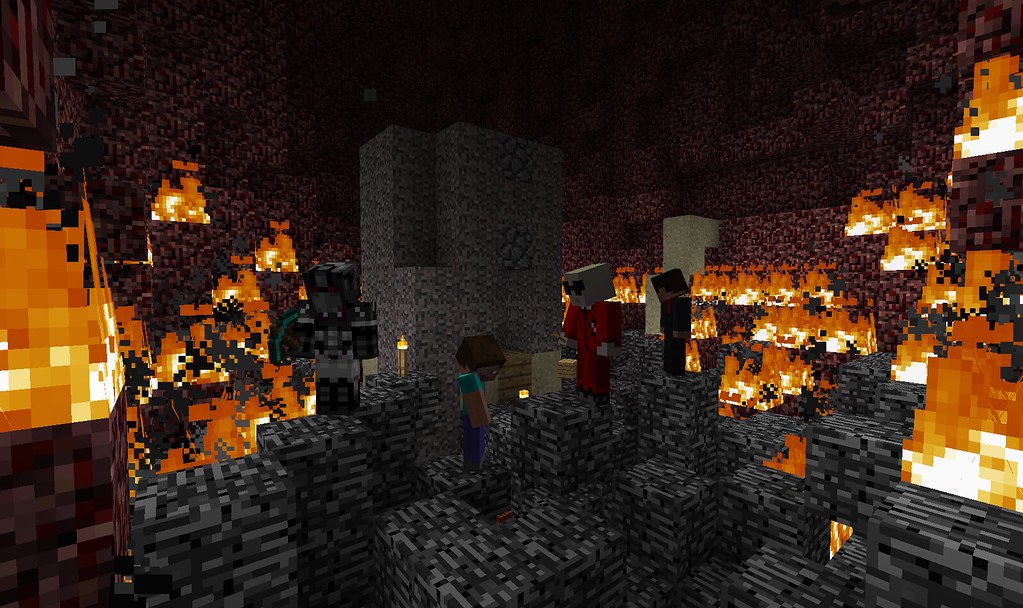The screenshot from Minecraft, captured in third-person view, features a group of four players situated in the Nether, the game's underworld. Three players showcase unique custom skins, while the fourth sports the default Minecraft skin, indicating they might be the one who captured the image. The scene is set at bedrock level, surrounded by netherrack and a significant pile of gravel. The environment is ablaze, suggesting the group might have established an operation or base in this perilous area. One player wields a diamond pickaxe, while the other three hold torches, each gazing in different directions, creating an enigmatic atmosphere as their exact activities remain unclear.